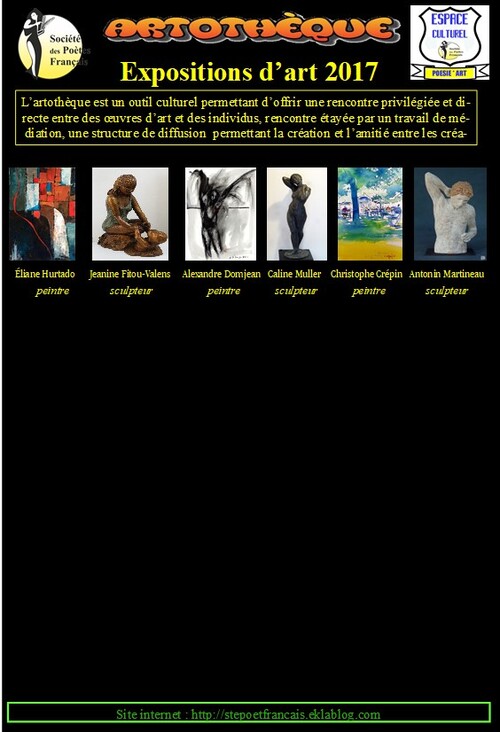This image features a detailed black background poster primarily focused on an art exhibition. Dominating the top of the poster, in large orange bubble letters, is the word "ARTOTHEQ." Immediately beneath it, in yellow text, is the subtitle "Exposition d'Art 2017." On the left side of the title, there's a circular emblem with an image of a person and the text "Societe de Poets Francais." To the right of the title, there's a small square containing the partially legible phrase "eSpace Cultural."

Directly below the main title, there is a text box with three lines of text in French, providing additional information about the exhibit. Beneath this text box, there are six small rectangles displaying photos of various artworks. Each photo includes yellow print descriptions below them, listing the artist's name and their medium. The artworks are: 

1. "Elaine Hurtado Pointre" 
2. "Jeanine Feteau Valens Sculpture"
3. "Alexandre Damjean Painter"
4. "Kaleen Muller Sculpture"
5. "Christophe Crepin Painter"
6. "Antoine Martineau Sculpture"

The depicted sculptures include a bronze statue of a woman seated on rocks, a nude figure on a pedestal with one arm behind its back, and a male torso with red hair, among others. The remainder of the poster, from the middle downwards, is a large black area devoid of any content. At the very bottom of the poster, highlighted in bright green, is the website URL: "Site Internet: http://stepoetfrancais.eclablog.com."